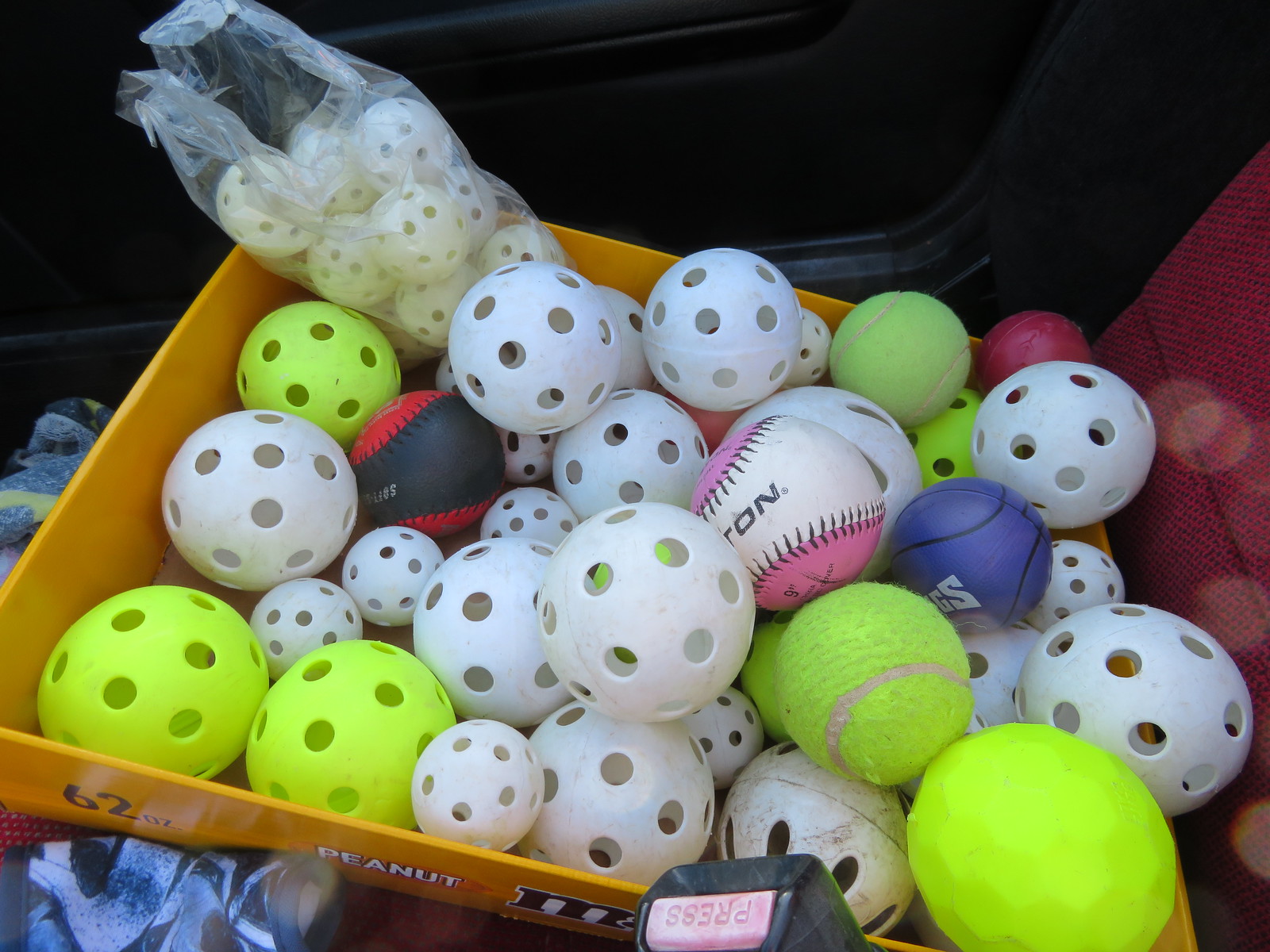The photograph features an eclectic assortment of balls, predominantly wiffle balls alongside several tennis balls and a single baseball. The collection is housed in a lidless M&M e-net box positioned on the passenger seat of a car with a reddish woven texture. Nestled inside the box are various sizes of wiffle balls, the majority of which are white, with some in bright yellow or neon green. A notable detail includes a bag of smaller, plastic-wrapped wiffle balls indicating their new condition. Additionally, the assortment includes a blue miniature basketball, and there appears to be a single softball and a black and red baseball. In the background, the interior of the car is partly visible, including a side door with a black interior and a blue shirt or blanket beneath the box.